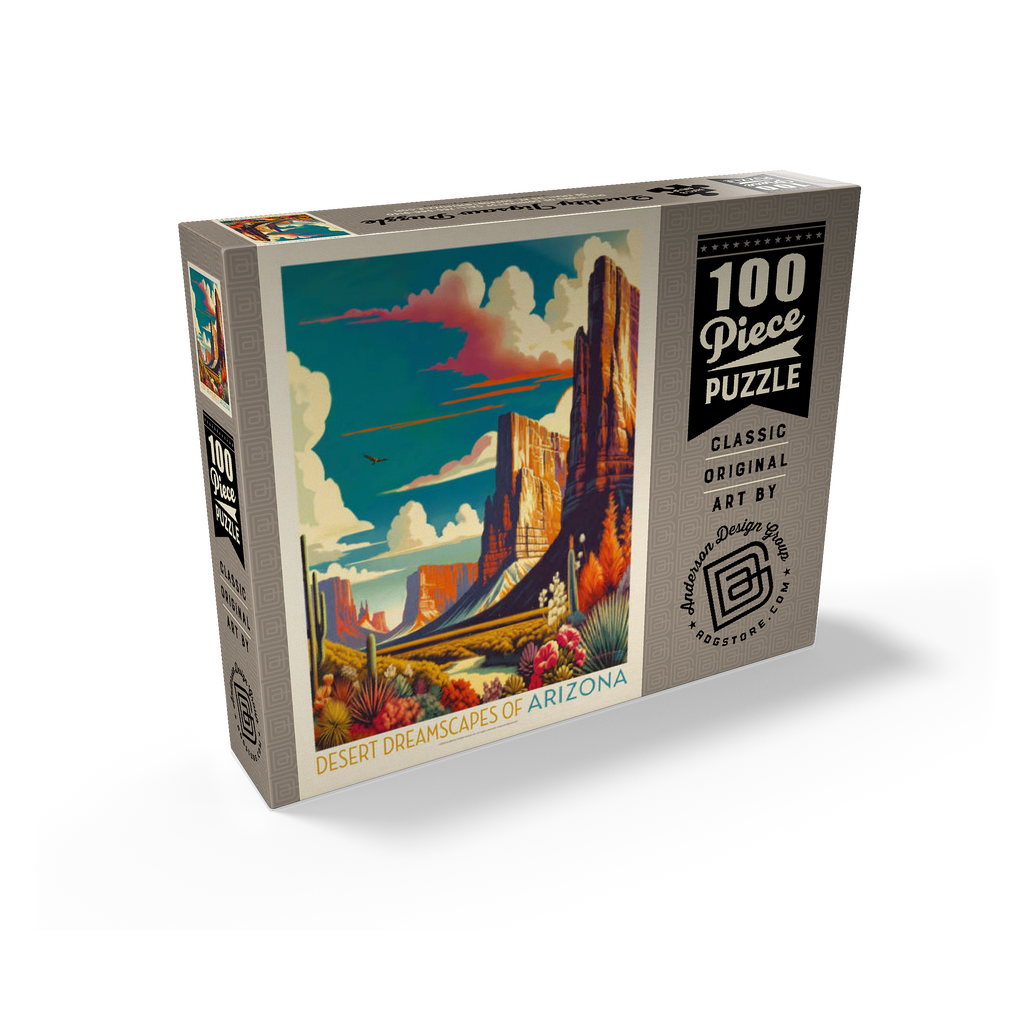The image displays a colorful box containing a 100-piece puzzle, titled "Desert Dreamscapes of Arizona." The box is predominantly gray with white and black text, and features a vibrant illustration reminiscent of a vintage 1950s postcard. This illustration, positioned on the front of the box, showcases tall mountains in shades of blue, green, yellow, and orange, with a blue sky and white clouds streaked with orange. A large bird is seen flying above the clouds. Below the mountains, the scene includes cacti, desert plants, flowers, and greenery, with what appears to be a wandering road or path through the mesas. The right side of the box bears a logo in a neutral taupe color reading "Anderson Design Group from adgstore.com," and a black ribbon banner denotes the puzzle's piece count, emphasizing its classic and original art design.